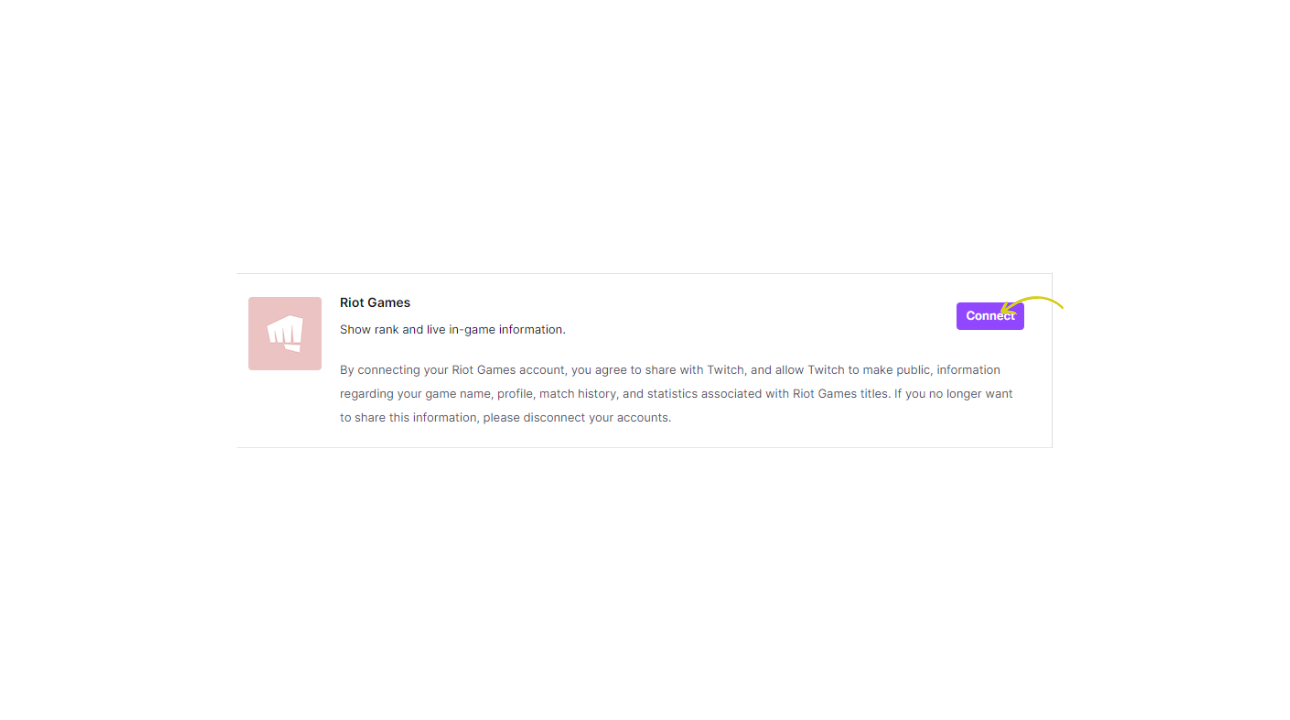The image displays a small rectangle outlined in a very light gray color. On the left-hand side, there is a prominent pink square featuring the image of a fist, with discernable fingers and a thumb, suggesting a symbol of strength or defiance. This square appears to display the text "Riot Games," although the text is somewhat unclear. Below this pink square, there is an additional line of smaller text that is not legible. 

Further below, there's another paragraph of text, even smaller and more difficult to read. To the right of the pink square, there is a purple rectangle containing a word that remains indiscernible. Superimposed on this purple rectangle is a yellow, curved arrow that extends towards the right-hand side of the image. The arrow seems to guide the viewer's attention from the text in the purple rectangle towards another part of the composition. 

All these elements are interconnected by a black line that is part of the light gray outline of the small rectangle. Once again, beneath the illegible lines of text appears the name "Riot Games," reinforcing the association with the gaming company. Despite the blurred text, the overall design suggests a structured layout with a focus on Riot Games and associated visual elements.